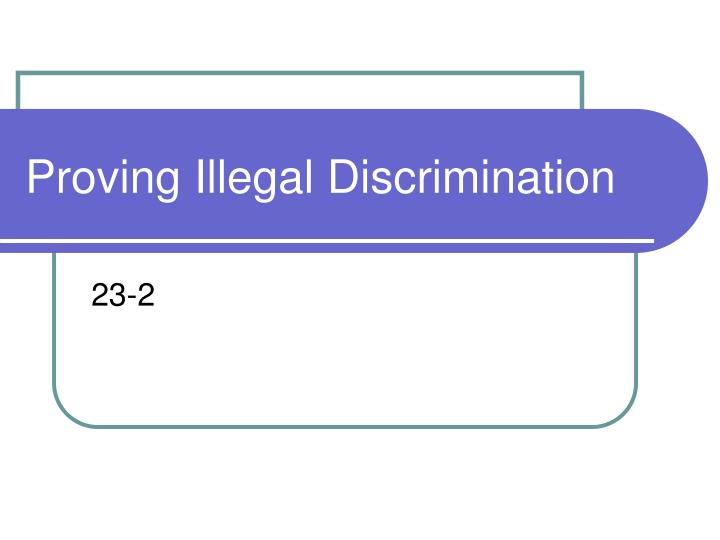This minimalist image, resembling a PowerPoint slide, features a central, light purple rectangle with rounded right edges and capped ends, making it half-circular on the right side. The focal point within this rectangle is the phrase "Proving Illegal Discrimination," displayed in white text, likely in a sans serif font. Running across the bottom of the purple rectangle is a thin white line. Surrounding this central element is a teal or green outline, creating a decorative border that continues above and below the purple rectangle. Below the main text, within this teal outline, is the black text "23-2." The overall layout is clean, with thin gray lines intersecting and providing a subtle frame for the image.